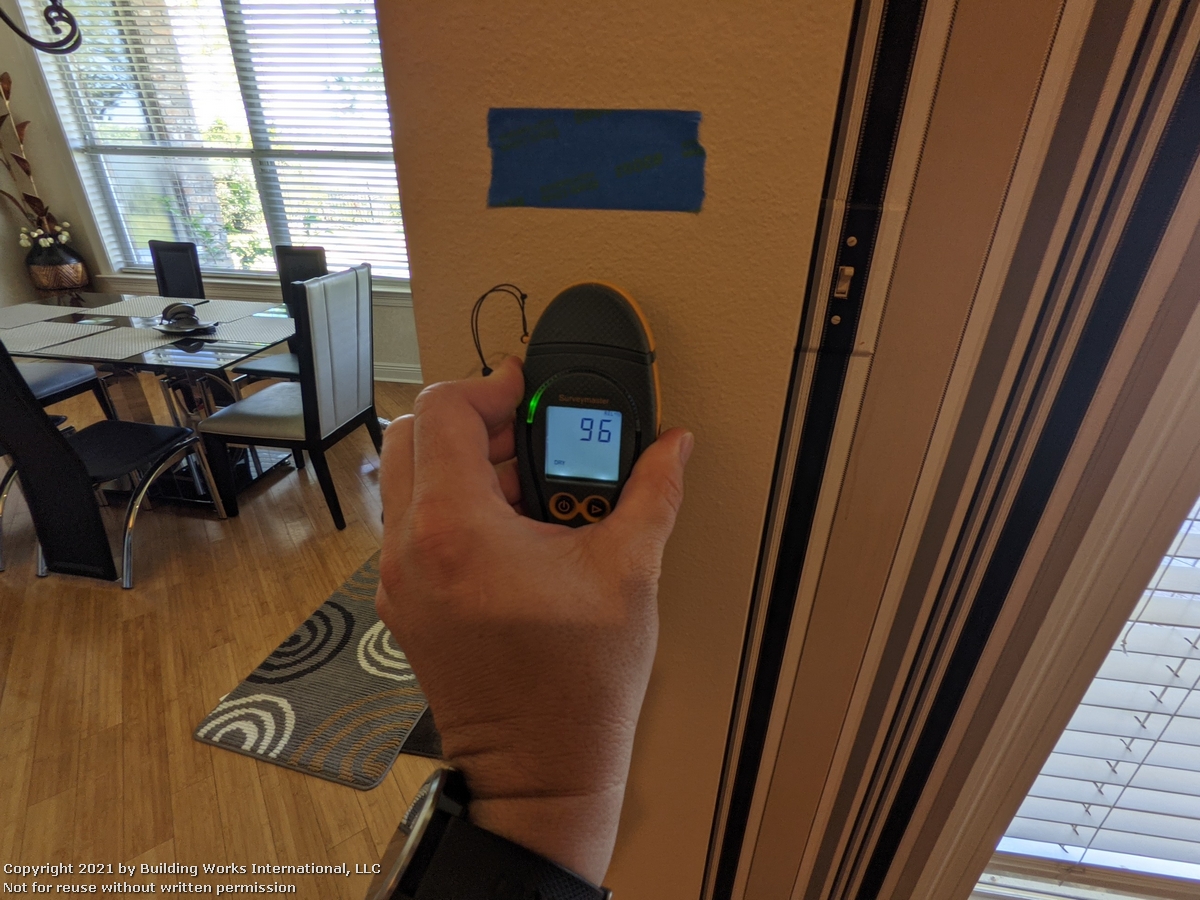The image captures a meticulously detailed interior of a room, emphasizing both the setting and an individual's interaction with a wall-mounted instrument. The focal point of the foreground is a man's left hand, adorned with a large wristwatch, as he operates or places a device displaying "96" next to a door frame. The device could be a phone or a thermostat and is mounted directly under a blue rectangular sticker. 

The room features a robust wooden floor with diagonal wood panels that prominently display their grain. Over the floor lies a grey rug embellished with white, black, and brown concentric circles. Positioned in the upper left section of the room, a glass dining table is surrounded by six leather chairs with black and white seats and metallic frames. The table is set before a window dressed with white Venetian blinds and features neatly arranged placemats, accompanied by an ornate brown and gold jug displayed in the corner. 

A second window, also adorned with white Venetian blinds, is visible on the right side of the image. The scene imbues a sense of sophistication and is further authenticated with a white-font watermark along the bottom left of the image, reading: "Copyright 2021 by Building Works International LLC, not for reuse without permission."